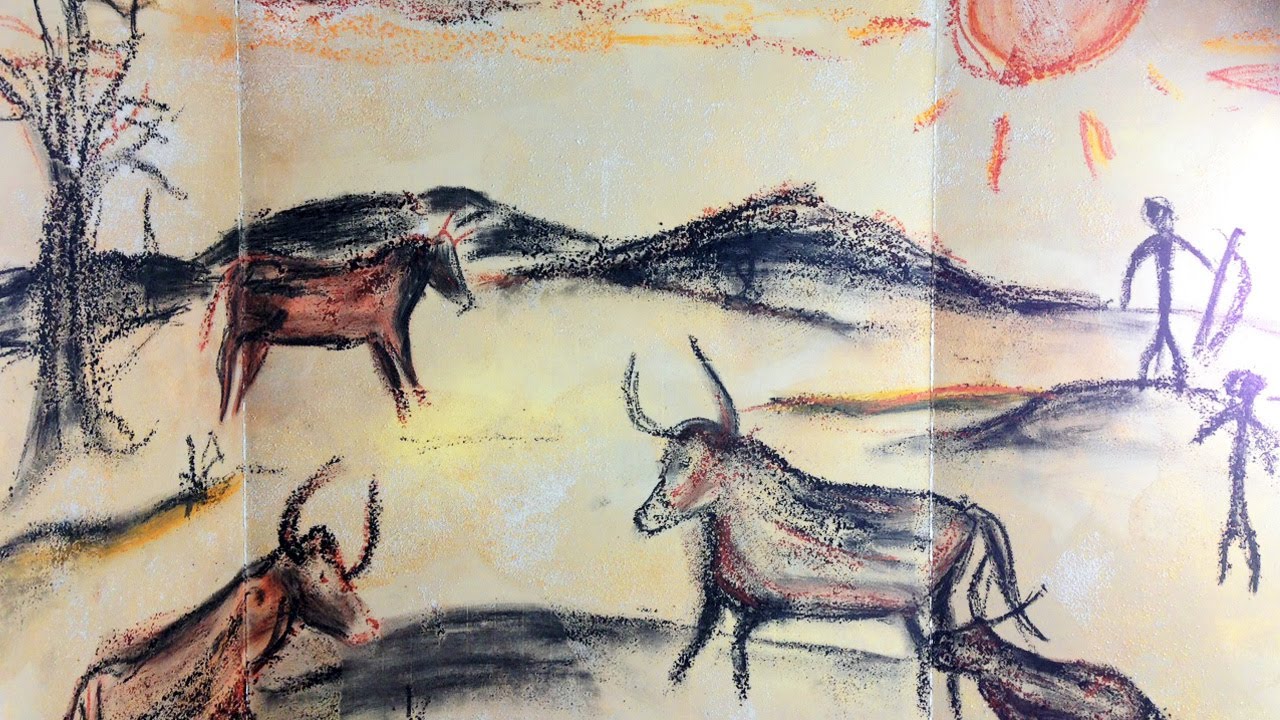The image resembles a child's crayon drawing on a wall, depicting a primitive hunting scene. There are two simple black stick-figure hunters, one standing on a small hill and holding a bow, while the other remains on the plains to the right of the image. The background displays a vivid landscape with dark gray mountain ranges, a leafless gray tree, and a light yellowish-brown land. At the top right corner, an orange sun with radiant rays lights up the scene, casting an orange hue through the sky. The central focus includes four bovine creatures, three large and one small, with details such as horns, tails, dark gray legs, and reddish-brown fur. Their varied positioning, with one facing the others across the bottom left, enriches the narrative, portraying a lively and dynamic hunt. The entire composition, through its simplistic yet vibrant crayon art, vividly captures the essence of an ancient hunting scene.